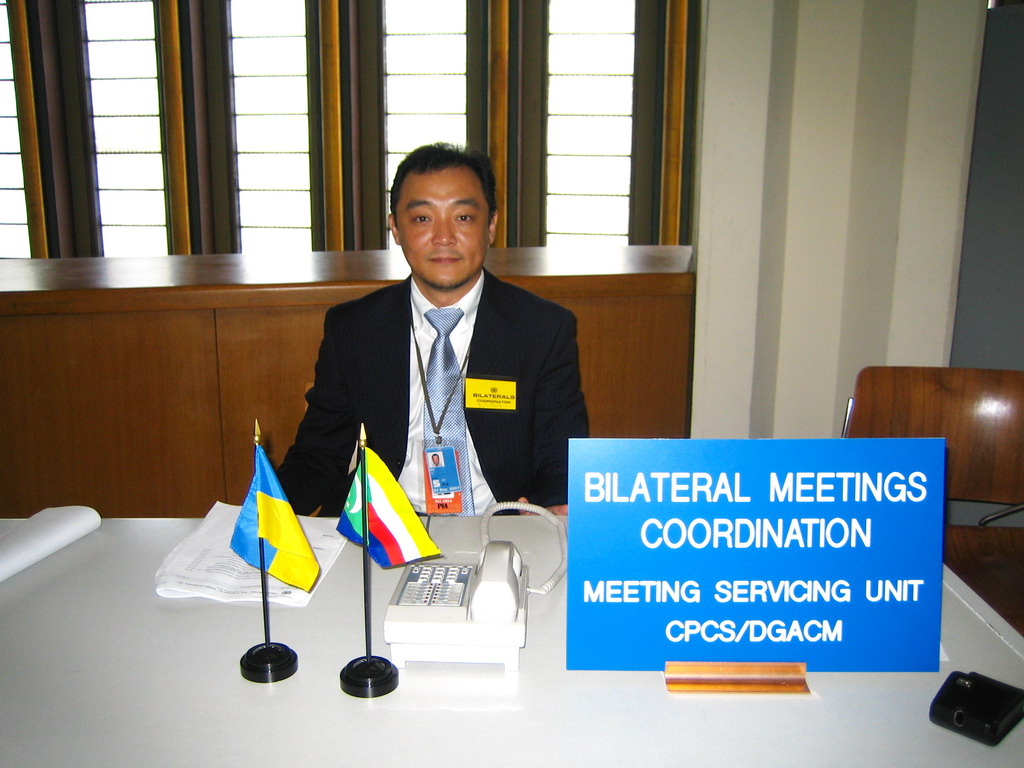In the image, an Asian man is seated behind a white desk, situated in a meeting room labeled with a prominent blue sign that reads "Bilateral Meetings Coordination Meeting Servicing Unit, CPCS DGACM." The gentleman is dressed formally in a dark blue suit complemented by a light blue tie and a white shirt. He wears credentials around his neck and has a yellow name tag pinned to his jacket. Behind him is a wall with windows that feature small openings, possibly segmented by five brown curtains, and there's a brown wooden cabinet adjacent to these windows. On the desk in front of him are a white touchstone phone, paperwork, a guest list, and a couple of small country flags positioned to the left. To the right of the desk, there's a school-style wooden chair.